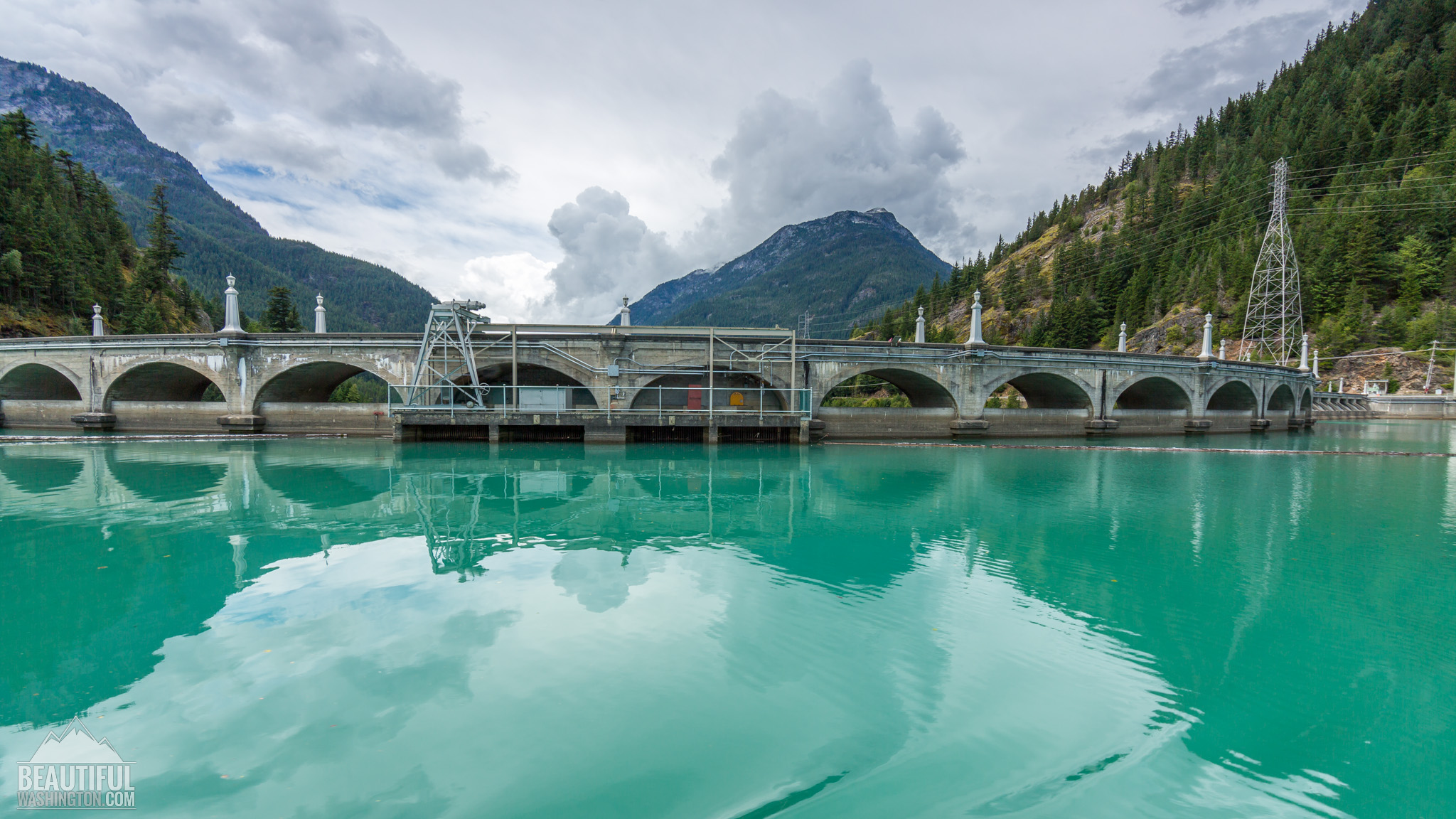The photograph captures a broad, sweeping view of a dam taken in the late afternoon under a predominantly cloudy sky with a few small patches of blue visible on the left. The backdrop features several tall mountains draped in a vibrant tapestry of green trees, emphasizing the grandeur of the landscape. The central focus of the image is the dam itself, a curved, imposing structure that holds back a body of water. The water in the foreground is a striking blue-green hue, reflecting the overcast sky and clouds above. The right side of the dam features an electrical tower. Intriguingly, a bridge-like structure with decorative arches and metal fencing, possibly scaffolding, juts into the water, adding an industrial touch to the otherwise natural scenery. Some text, partially obscured, is visible in the bottom left corner of the image, hinting at an unknown website.